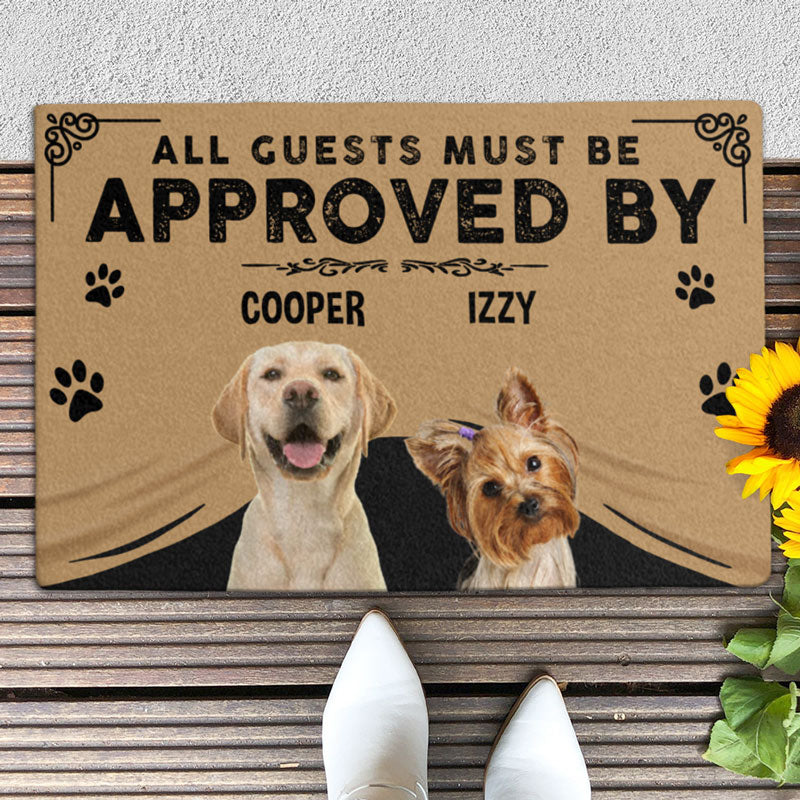The image features a custom-designed doormat with a whimsical, tongue-in-cheek message that reads, "All guests must be approved by Cooper and Izzy" in bold black lettering. Pictured on the mat are two friendly-looking dog portraits: Cooper, a Labrador Retriever, with an open-mouth smile, and Izzy, a Yorkshire Terrier adorned with a purple bow in her hair, tilting her head inquisitively. The dogs appear to be peeking out from under a brown curtain-like fabric, creating the illusion that they are emerging from beneath the doormat. Flanking the text are dark brown paw prints, adding a playful touch. The mat itself rests on wooden slat flooring, and the tips of someone's white shoes are visible at the bottom. Adjacent to the mat on the right is a partially visible bright yellow sunflower. The doormat, with its light brown background, includes intricate details, such as the illusion of the mat being slightly lifted where the dogs appear, making the overall design both charming and engaging.